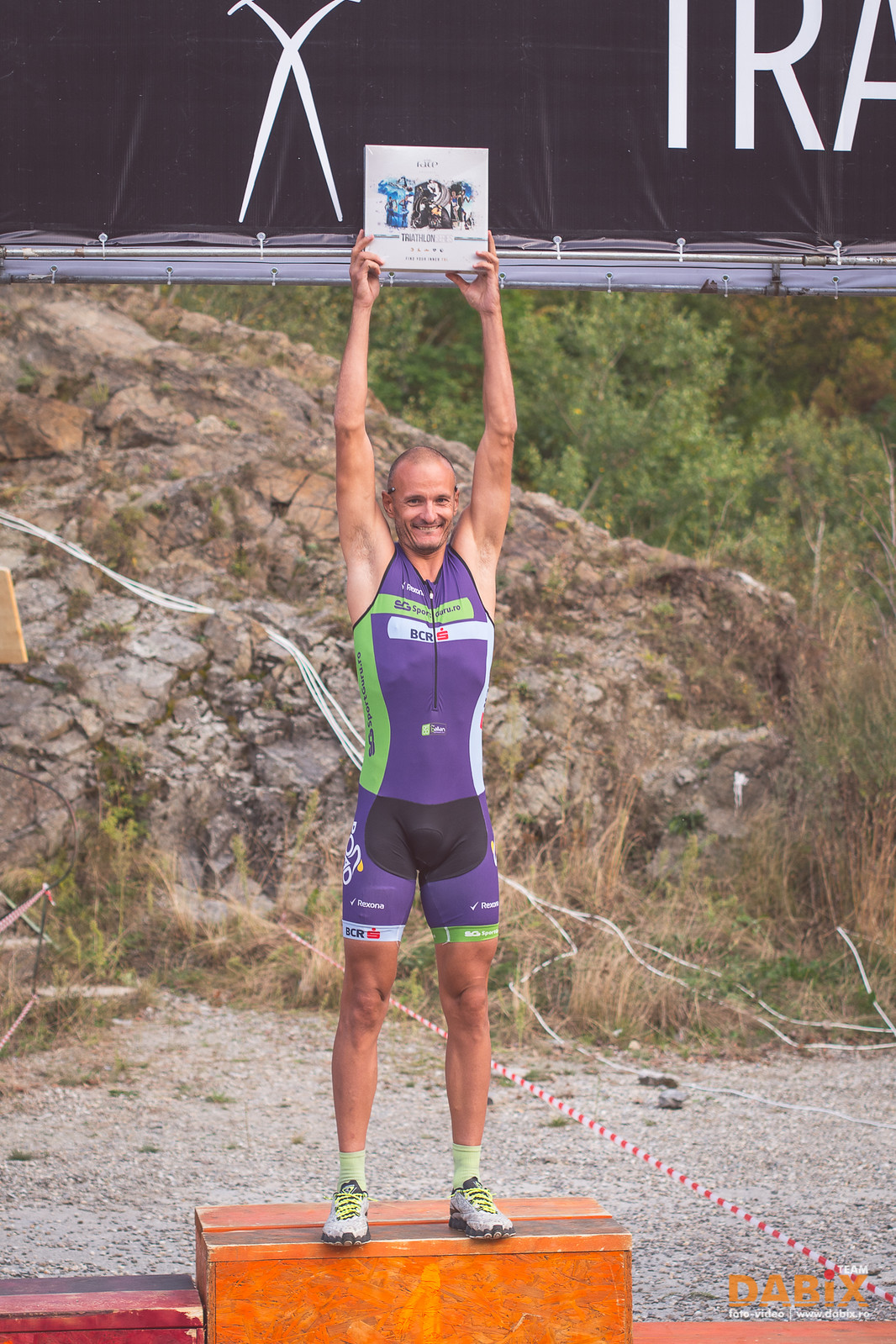This detailed photograph, taken outdoors, captures a triumphant runner standing at the center of the image on a wooden first place podium, which has a yellow to orange hue. Flanked by smaller pedestals on either side, the runner stands tall, raising a white square sign above his head that displays some colorful images, possibly t-shirts, though it's difficult to discern due to the distance. He is attired in a distinctive one-piece athletic tracksuit predominantly colored in shades of purple, blue, green, and black with green trim, sleeveless and cutting off at the upper thighs. The suit features a zipper down the middle. His light green or gray shoes with yellow laces complement his green socks. The runner sports a huge smile and a shaved head, signifying a victorious moment likely after a triathlon.

In the background, the setting reveals a gravel lot extending into a rough, uphill terrain with rocks and weeds, and green bushes scattered around. Beyond this, a line of trees is visible, indicating a natural, rugged landscape. Hanging above the runner is a partially visible black banner inscribed with white text and a criss-crossing X logo, adding an official touch to the scene. The combination of natural elements and race paraphernalia creates a compelling snapshot of the celebratory moment.